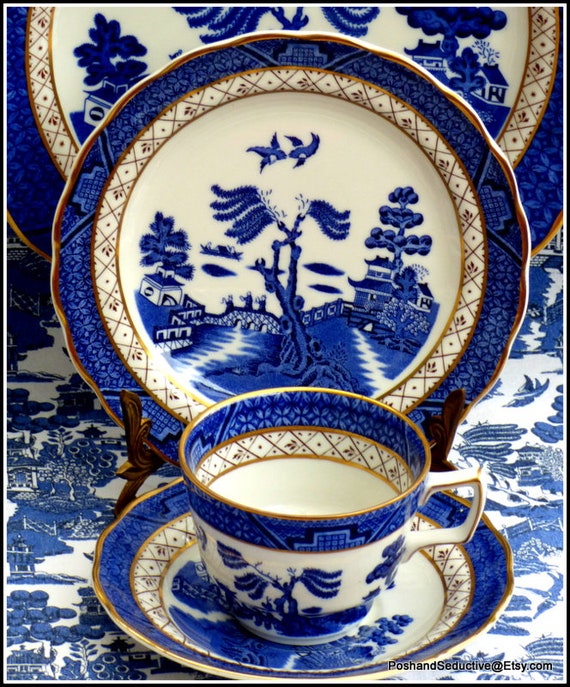The image showcases an elegant china set arranged on a tablecloth that shares a complementary pattern and color scheme. The set consists of four pieces: a large plate, a smaller plate, a saucer, and a teacup. Each piece features a harmonious palette of white, blue, and gold. The gold trim elegantly lines the edges, including the rim of the teacup and the inner curves of the plates, accentuated with a diamond pattern. 

The designs on the china depict serene scenes of trees, oriental-style houses, and birds, adding a picturesque touch to each item. The smaller plate, prominently placed at the center, displays a detailed vignette with a whole tree, two birds mid-flight, and multiple houses. The teacup, resting on its matching saucer in front of the smaller plate, also features intricate imagery of trees on its exterior, while the inner side showcases the blue and gold color scheme.

In the background, a large plate partially obscured, still reveals glimpses of the depicted trees and houses, adding depth to the arrangement. The collection is presented on a tablecloth that mirrors the blue and white tones of the china, enhancing the cohesive aesthetic. 

In the bottom right corner, the text "POSH and Seductive at Etsy.com" suggests that this image may serve as an advertisement, possibly for a handcrafted or curated collection available for purchase.